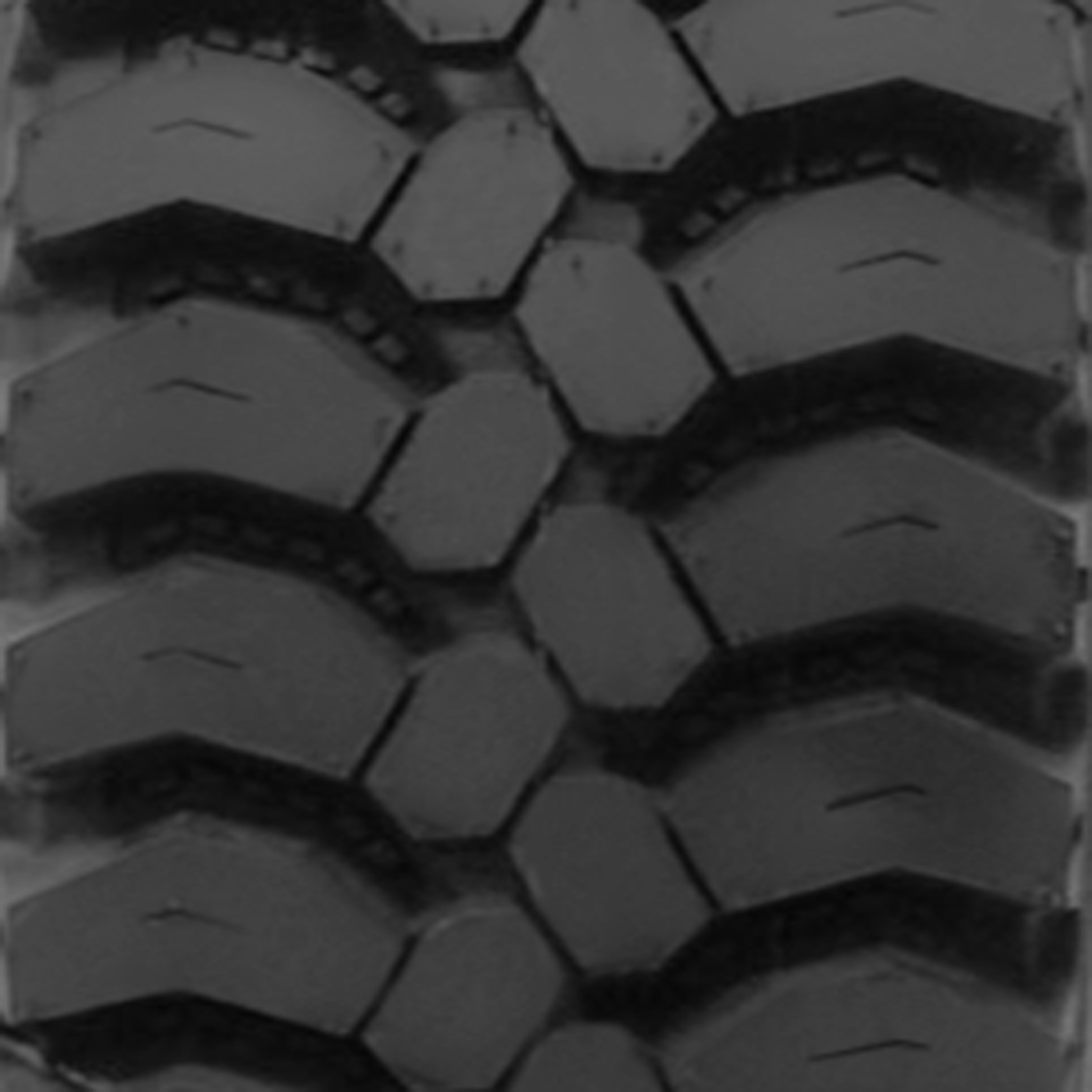This is a square image depicting a highly magnified, low-resolution close-up of what appears to be multiple brake pads arranged against a white background. The image is primarily in shades of black and gray, with two rows of brake pads: four on the left and five on the right. The brake pads feature small notches on their top side, cupping over the pad, and additional notches in their centers. The geometrical shapes and lines in the image could be mistaken for the tread of a tire due to their intricate and patterned design. The darkened shadows between the grooves of the black rubber-like material add depth to the image, which lacks any distinct background, making the array of shapes the focus of the photograph.